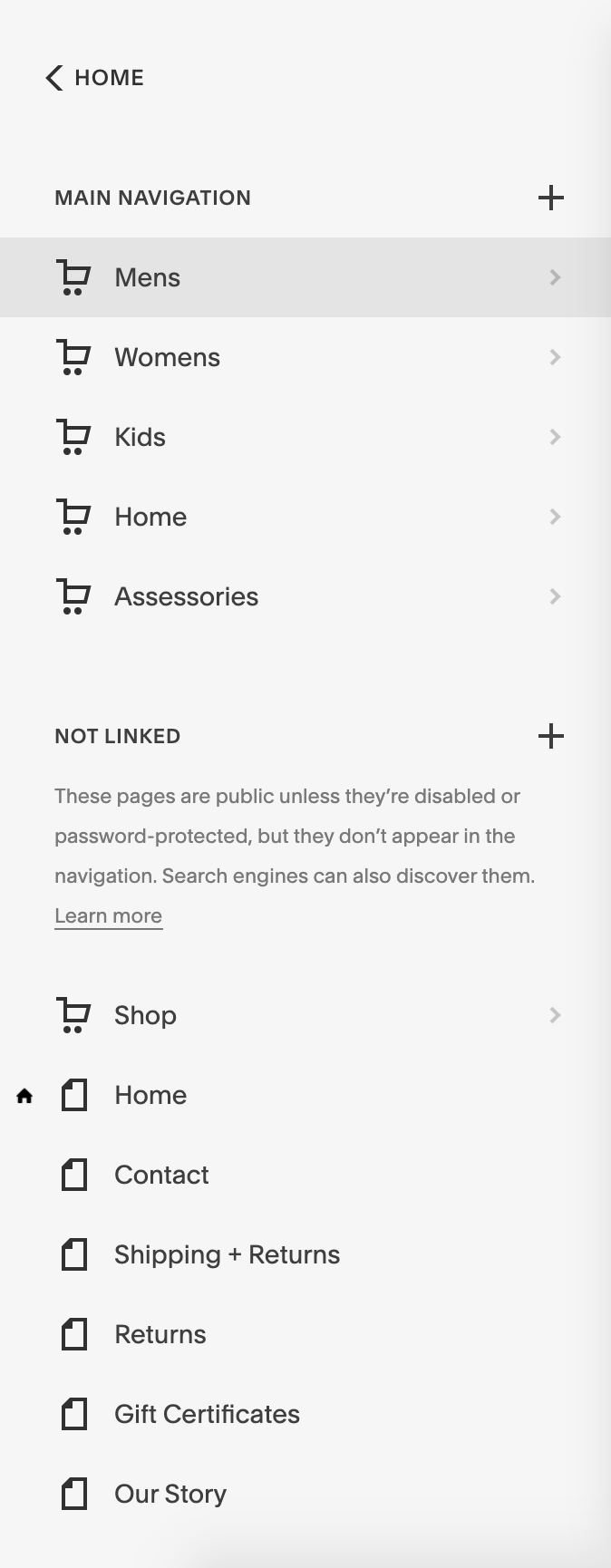Screenshot of a mobile app displaying a grey-themed menu navigation interface. At the top of the screen, there is a header labeled "Home," accompanied by a 'Go Back' button on the left-hand side. Below this, the title "Main Navigation" is displayed with a plus icon for expanding the menu. The options listed under this section include "Men's," "Women's," "Kids," "Home," and "Accessories," each with a stylized shopping cart icon on the left and a right-pointing arrow on the right to reveal further sub-menus.

Further down, another header reads "Not Linked" followed by a plus button to expand this section. It indicates that these pages are public unless disabled or password-protected, and notes that search engines can discover them, with a clickable underlined "Learn More" link for additional information. 

The vertical menu continues with sections labeled "Shop," "Home," "Contacts," "Shipping and Returns," "Returns," "Gift Certificates," and "Our Story." Each entry is accompanied by an appropriate icon: a shopping cart icon next to "Shop" and a home icon beside "Home." The remaining items ("Contacts," "Shipping and Returns," "Returns," "Gift Certificates," and "Our Story") each feature a dog-eared page icon to their left. The "Shop" entry, like some previous categories, includes a right-pointing arrow to explore additional sub-options.